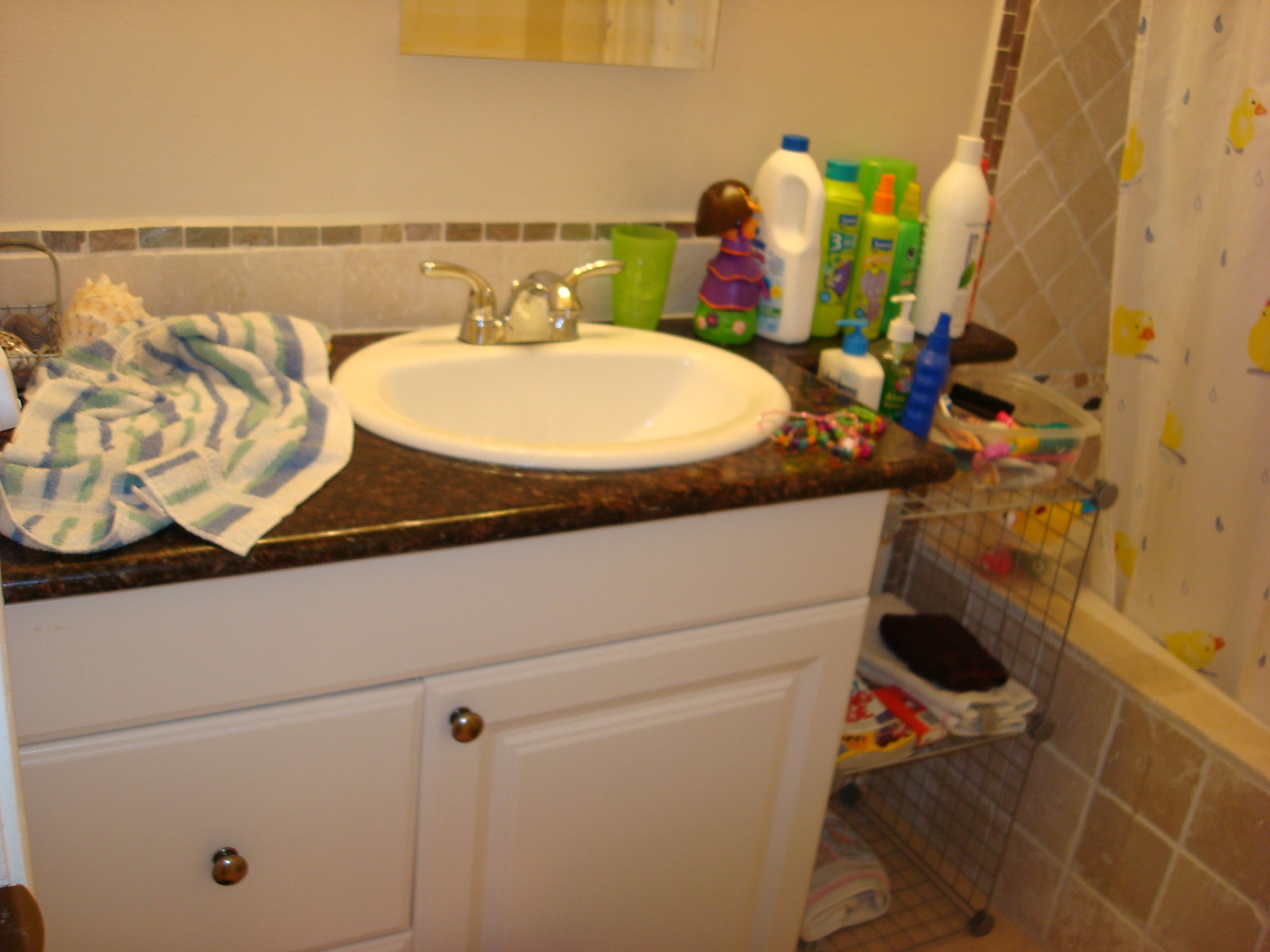The image depicts a somewhat blurry photograph of a bathroom with notable details. On the left side, a white cabinet stands out with its shiny wooden countertop, adorned with a pristine white sink and sleek silver fixtures. The cabinet features at least two drawers on the left and a cabinet door on the right. Draped over the left side of the sink is a rumpled towel, patterned with blue, green, and white stripes. Various hair products are neatly arranged nearby.

Adjacent to the sink is a wire shelving unit. The bottom shelf holds a towel, while the second shelf has a stack of neatly folded towels. The upper shelves feature a collection of items, including a white bottle with a blue lid, a green liquid bottle resembling hand soap, and a clear container filled with miscellaneous objects. To the right, there is a light brown tiled shower and bath combo, complemented by a clear shower curtain decorated with playful duck illustrations.